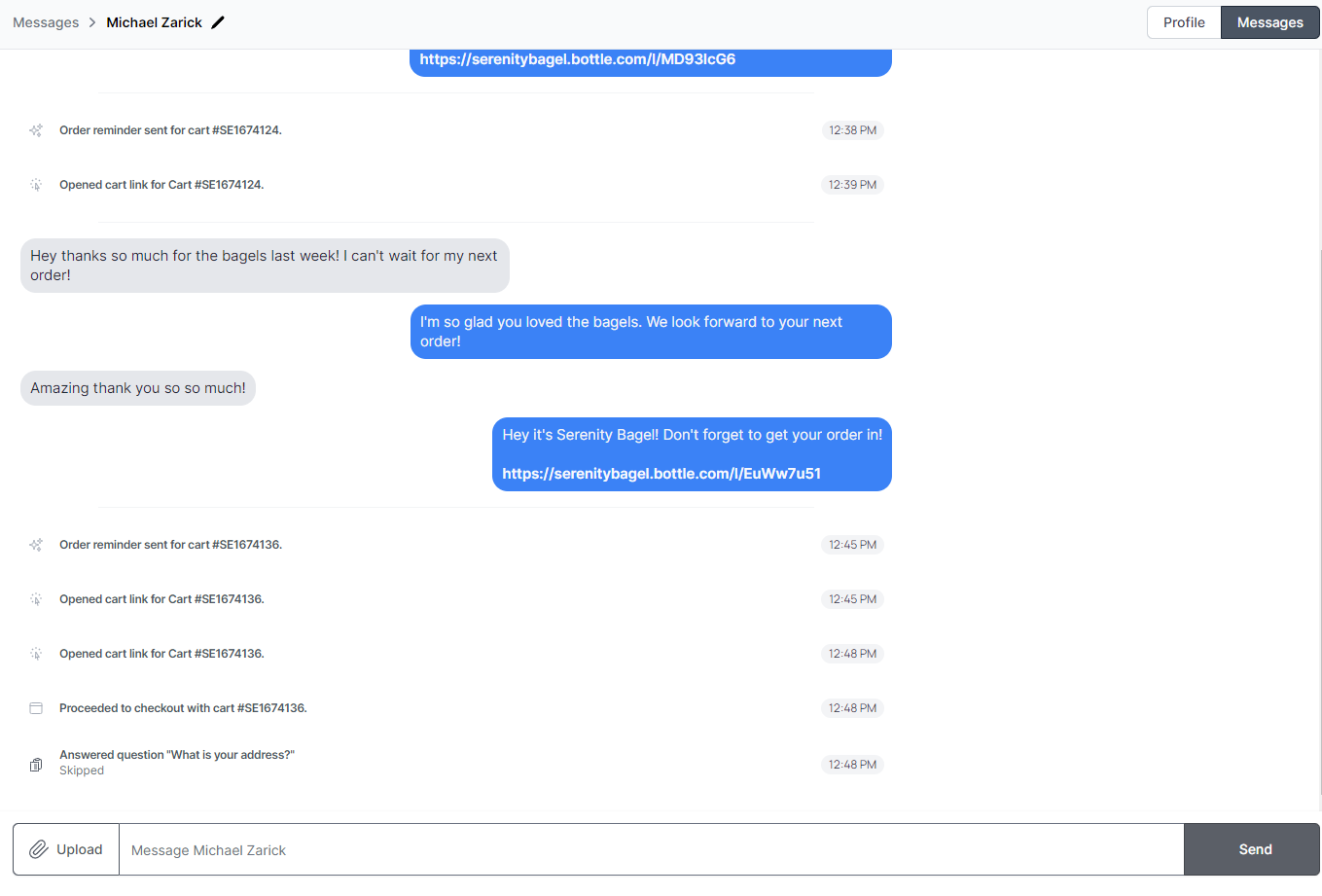Here is a detailed and cleaned-up caption for the given image:

---

This screenshot displays a messaging interface, potentially from a phone, website, or app. In the upper left corner, the title "Messages" appears, accompanied by the name "Michael Zarek" and a small black pen icon. The upper right corner features two clickable buttons: "Profile" with a white background and "Messages" with a gray background. The main screen showcases a series of messages exchanged between users.

1. The first visible message reads, "Order reminders sent for cart number SE 1674124 at 12:38 PM."
2. Following this, another message states, "Open cart link for cart number SE 1674124 at 12:39 PM."
3. The subsequent interaction includes informal conversation, starting with a message that says, "Hey, thanks so much for the bagels last week. I can't wait for my next order."
4. The response to this message reads, "I am so glad you love the bagels. We look forward to your next order."
5. Continuing the conversation, another message says, "Amazing, thank you so much!"
6. Then, a promotional message from Serenity Bagel follows: "Hey, it's Serenity Bagel. Don't forget to get your order in," accompanied by a link, "http://SerenityBagel.bottle.com/i/EUWW7U51."
7. Below this, the message thread includes a series of order and pickup reminders.

At the bottom of the screen, there is a message input bar with a "Send" button located in the bottom right corner.

---

This caption provides a clear, comprehensive description of the content and layout of the messaging interface shown in the screenshot.